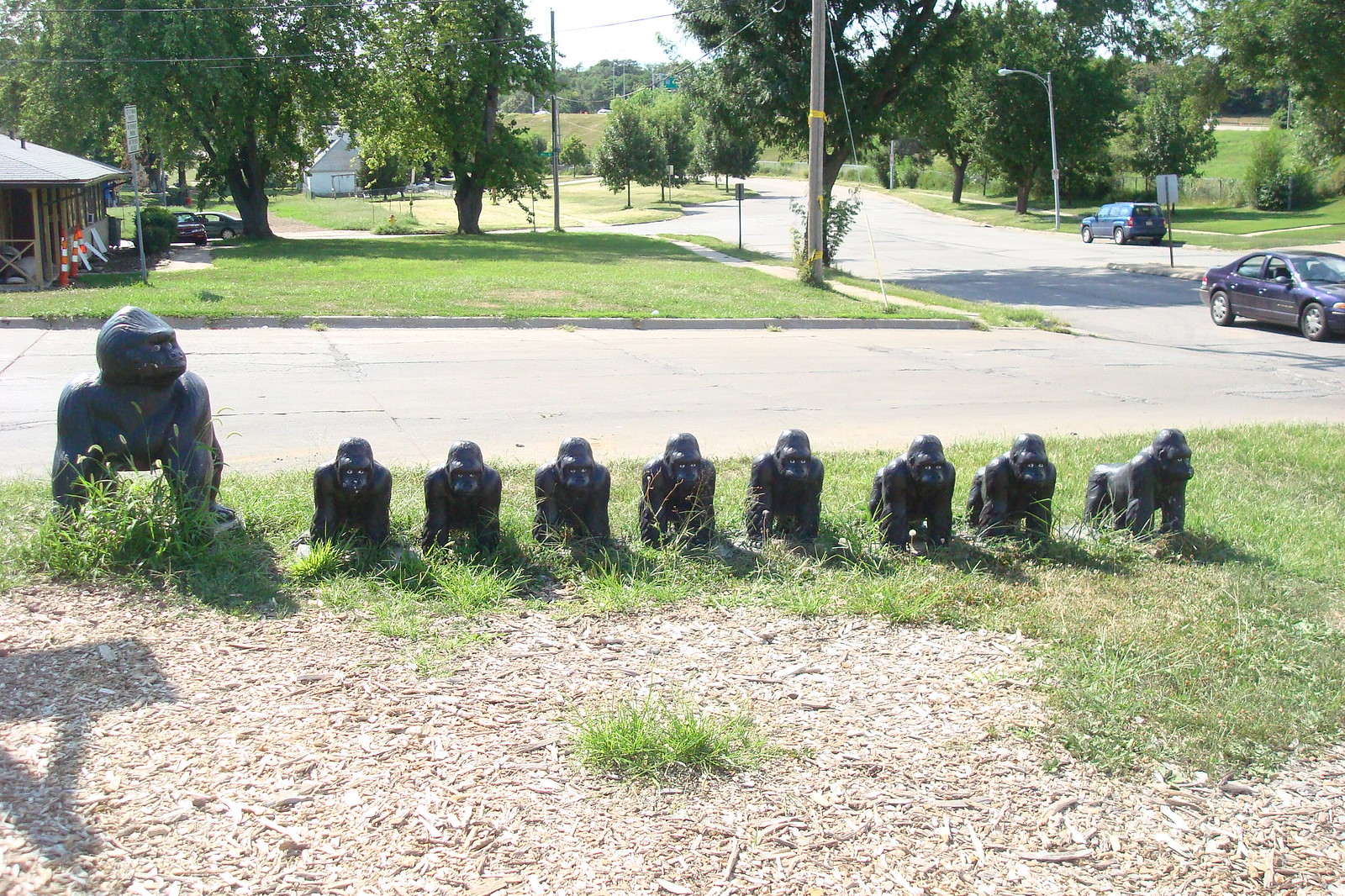This is a horizontal rectangular color photograph capturing a scene with nine gorilla statues arranged on a patch of weedy green grass interspersed with landscaping wood chips. Eight smaller gorillas crouch on all fours in a downward position across the middle of the frame, while one much larger gorilla on the far left mirrors their pose. The smaller statues appear to be facing straight ahead or slightly to the lower right, with intent expressions directed towards the viewer, while the larger gorilla seems to be gazing at the middle-right side of the image. Behind them, a road runs horizontally with a dark-colored car cut off on the right side and another vehicle, possibly an SUV or minivan, moving away towards the top middle of the photo. The backdrop features a rural or suburban setting with grassy expanses, numerous trees, and buildings including a brown structure with a patio to the left, cars parked in front of it, and another light-colored building further in the background. The scene is well-lit, suggesting a sunny day.